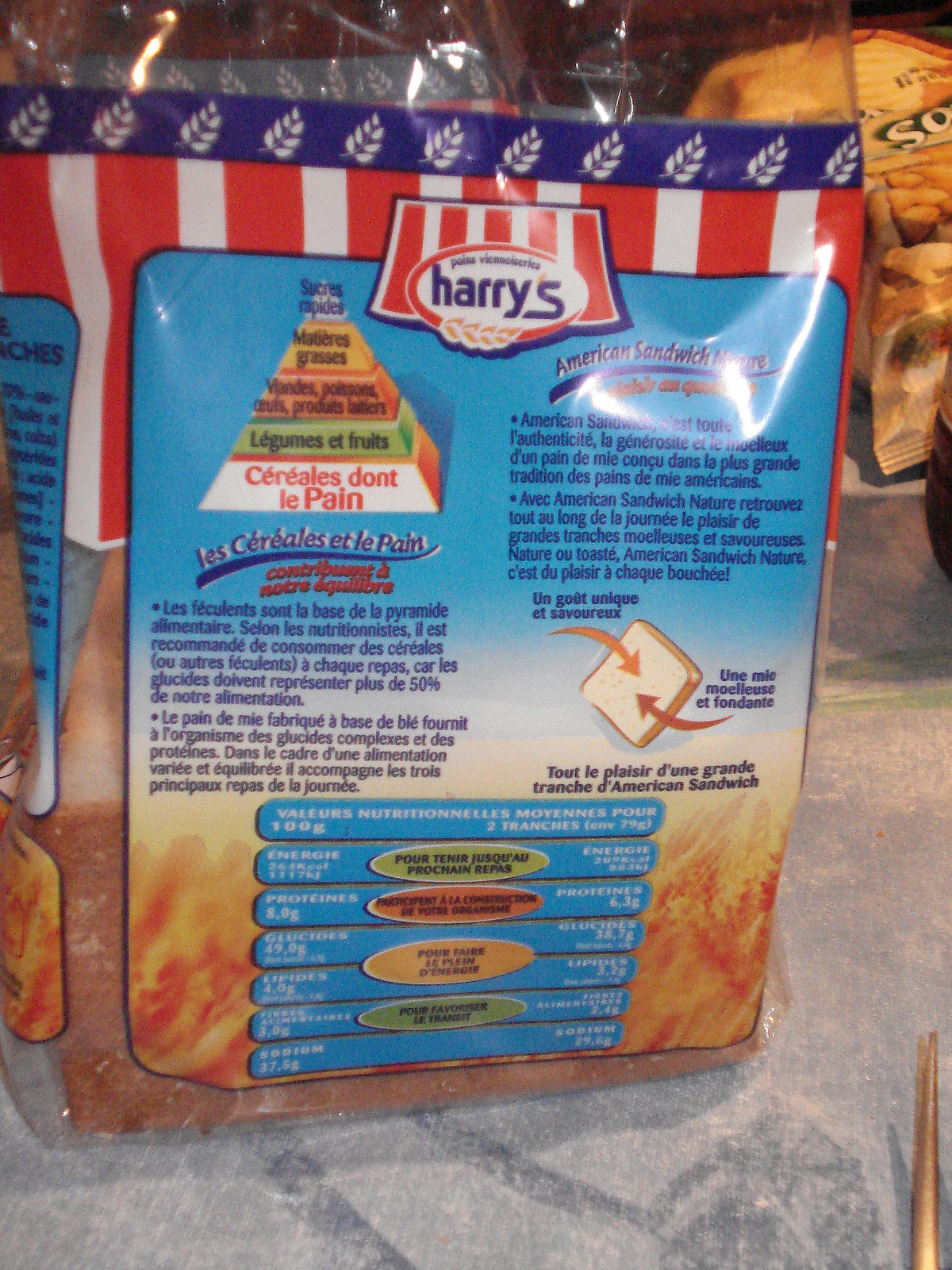In the background of the image, there is a bag of food that prominently displays the brand "Harry's." The text on the bag suggests that it contains bread, labeled as "American Sandwich." The packaging has a noticeable shine, likely from the camera flash, giving it a slight glow. Additionally, the bag features text in French, which reads "Les Céréales et le Pain" translating to "The Cereals and the Bread."